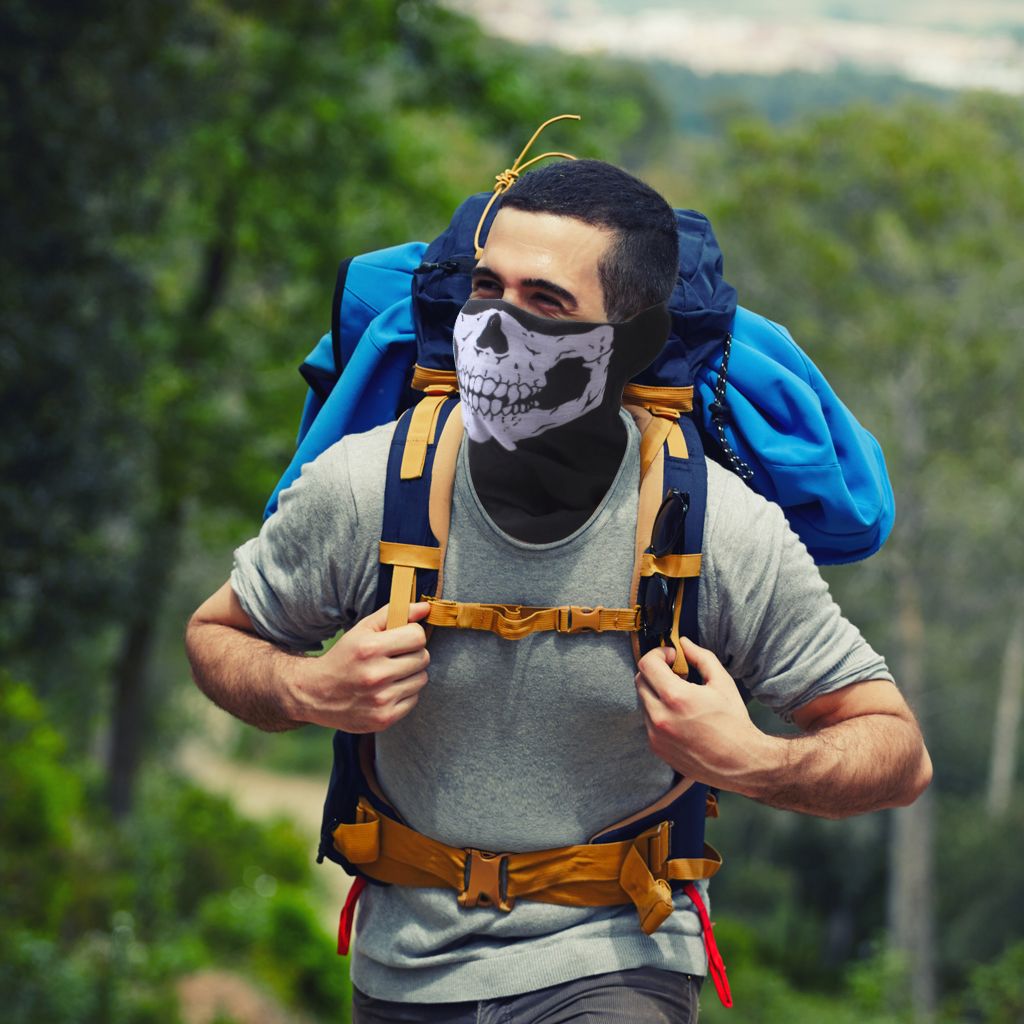In the image, a solitary hiker is captured in a vibrant woodland setting, characterized by lush green trees and plants, with possible waterfalls subtly visible in the bottom right corner. The man, dressed in a gray t-shirt and gray pants, carries a conspicuous blue backpack with multiple colorful straps—yellow, orange, and tan. The backpack appears very full, with what seems to be a sweatshirt or blanket protruding from either side. Notably, he's wearing a strikingly eerie mask with a skeleton's face painted on it, reminiscent of those worn during the COVID pandemic. This mask, blue with a skull design covering his mouth and forehead areas, adds an unusual, almost haunting element to the scene. His backpack is equipped with red pull strings at the bottom and black sunglasses secured to the front. The hiker's hands rest on the straps of his backpack, and despite the somewhat unsettling mask, he appears to be enjoying his outdoor adventure. The background blurs slightly, enhancing the focus on the hiker while also hinting at the serene, expansive wilderness surrounding him.